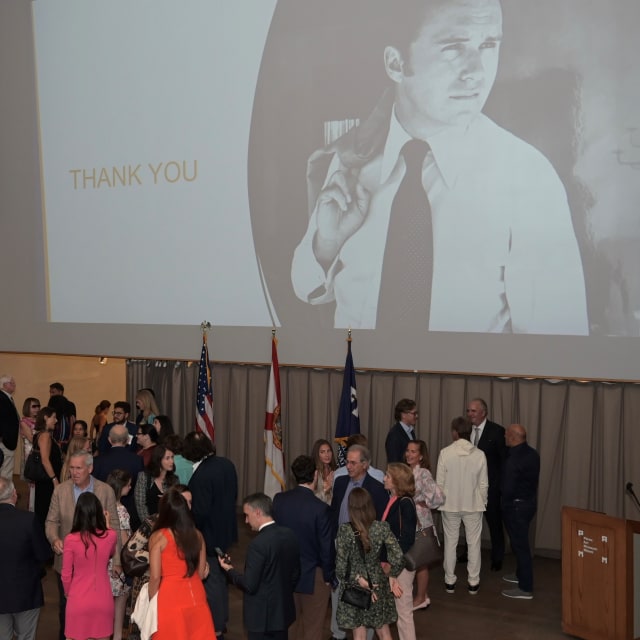The image captures a formal gathering set on a stage, with elegantly dressed attendees in suits and dresses scattered across a dark floor. Dominating the scene is an enormous projector screen displaying a black and white image with the words "thank you" prominently in gold. The screen also features a man dressed in a long-sleeved white dress shirt and dark tie, holding a jacket over his shoulder in a model-like pose. In the bottom left corner, a lady in an orange dress stands beside another in pink. To the right of the screen, towards the middle, a wooden podium is visible, bearing a square plaque and a black microphone. Additionally, three flags—one American and two unidentifiable due to being partially folded—are propped against the front of the room. It appears to be a sophisticated event, with guests engaged in conversation and socializing in a business casual setting.